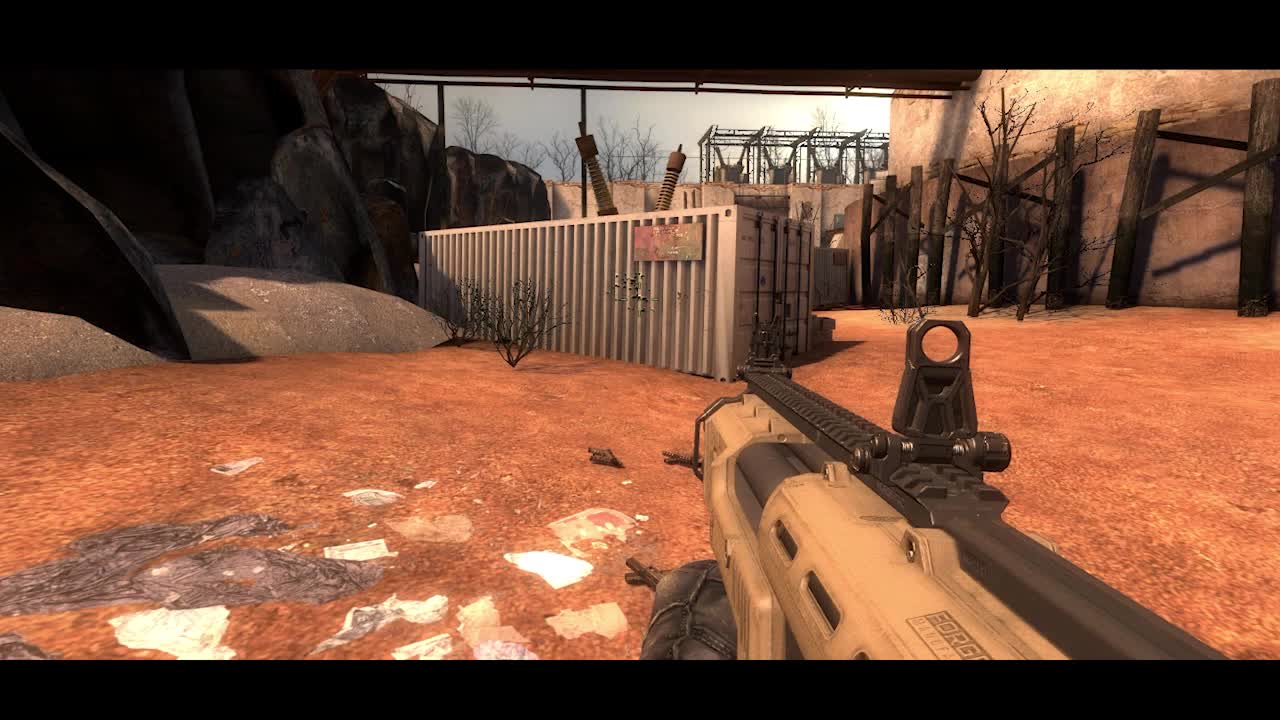The image captures an outdoor scene from a first-person shooter video game, set in a seemingly desolate, sandy environment with a rust-colored ground indicative of a desert setting. Dominating the background is a large, tan stucco wall, alongside which stands a wire mesh structure. To the right, another building features the same stucco material, in front of which several wooden boards are vertically positioned against the wall with some scattered twigs. Centered in the scene is a large crate or cart, possibly metal or plastic, topped with protruding screws. A distinctive long barrel of a rifle is pointed directly ahead, emphasizing the first-person shooter perspective. Additionally, the background includes a sky that is blue with patches of white, and there is a small leafless tree beside the crate, reinforcing the abandoned, rugged atmosphere of the setting.